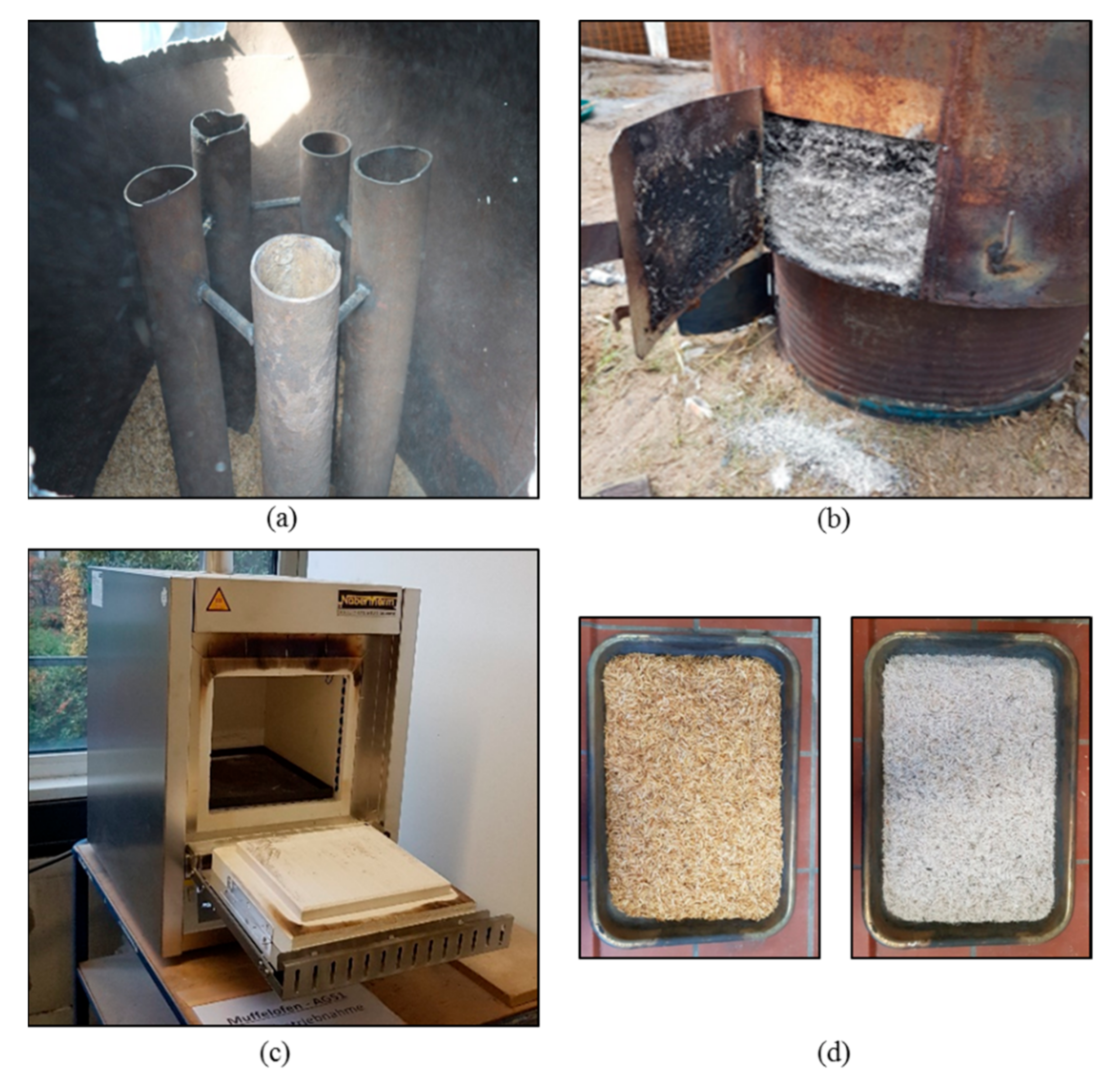The image is a square grid divided into four labeled segments: A, B, C, and D. Segment A, located on the top left, features five cylindrical pipes in shades ranging from light gray to dark gray, arranged vertically within a grey enclosed space. Segment B, on the top right, depicts an extremely dusty, rusted cylindrical object resembling an old water heater or oil burner positioned in the upper right corner on a dirt ground, complete with ridges and a small door at the bottom. Segment C, found on the bottom left, is a smaller silver appliance that looks like an oven with its door open, exposing a charred interior, set on a countertop. Finally, Segment D, on the bottom right, shows two rectangular trays, one filled with brown granules that resemble wood chips or brown rice, and the other with white granules akin to ash or white rice. The four images together evoke a transition from old, potentially incinerated items to what may be their resulting ashes, forming a thematic collage.